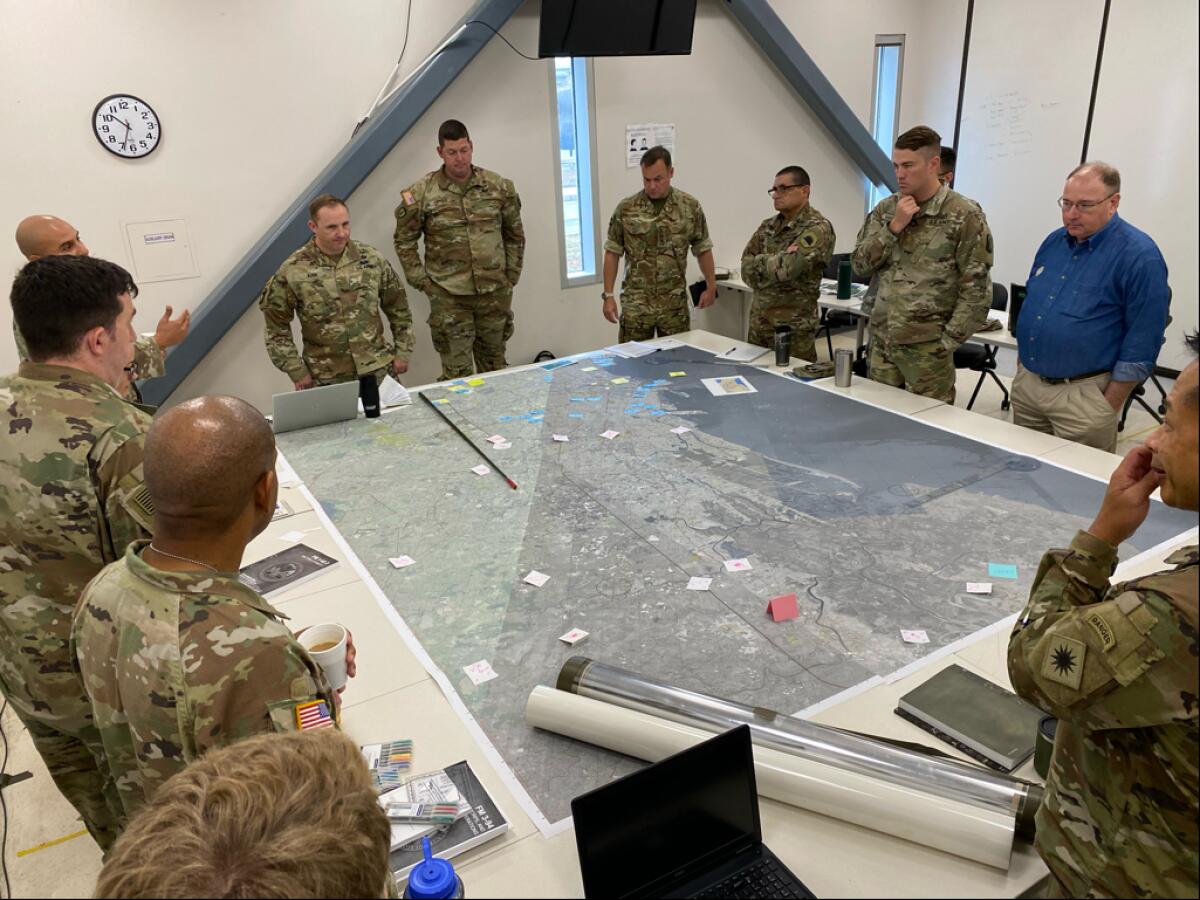The photograph captures an intense scene inside a modern war room, with a focus on a large, rectangular conference table dominating the center. Spread across the table is an expansive reconnaissance map, detailed with aerial views and strewn with numerous sticky notes, suggesting meticulous planning. The room is markedly professional, its white walls punctuated by narrow vertical slit windows that allow natural light to pour in, highlighting the seriousness of the ongoing discussion.

Gathered around the table are eleven men, predominantly in US Army camouflage uniforms, with one notable civilian in a denim shirt and khaki pants. This civilian, distinguishable by his glasses, is out of place among the trim, military-fit officers. To his right stands a South Asian man whose left arm bears a tan patch marked with a black starburst emblem. An African-American officer with a shaved head, dog tag chain barely visible at the back of his neck, clutches a styrofoam coffee cup in his left hand, while the top of a Nalgene water bottle peeks out from the lower left corner of the image.

The meeting appears highly strategic, underscored by the presence of two laptops, additional coffee cups, a rolled-up map, and a pointing stick. A wall clock reads 6:50, and judging by the brightness outside, it could very well be in the morning. The officers, identifiable by US patches on their right arms, are deeply engaged in what looks like an intense deliberation over the maps, likely planning a crucial operation reflected by the detailed reconnaissance material spread before them.